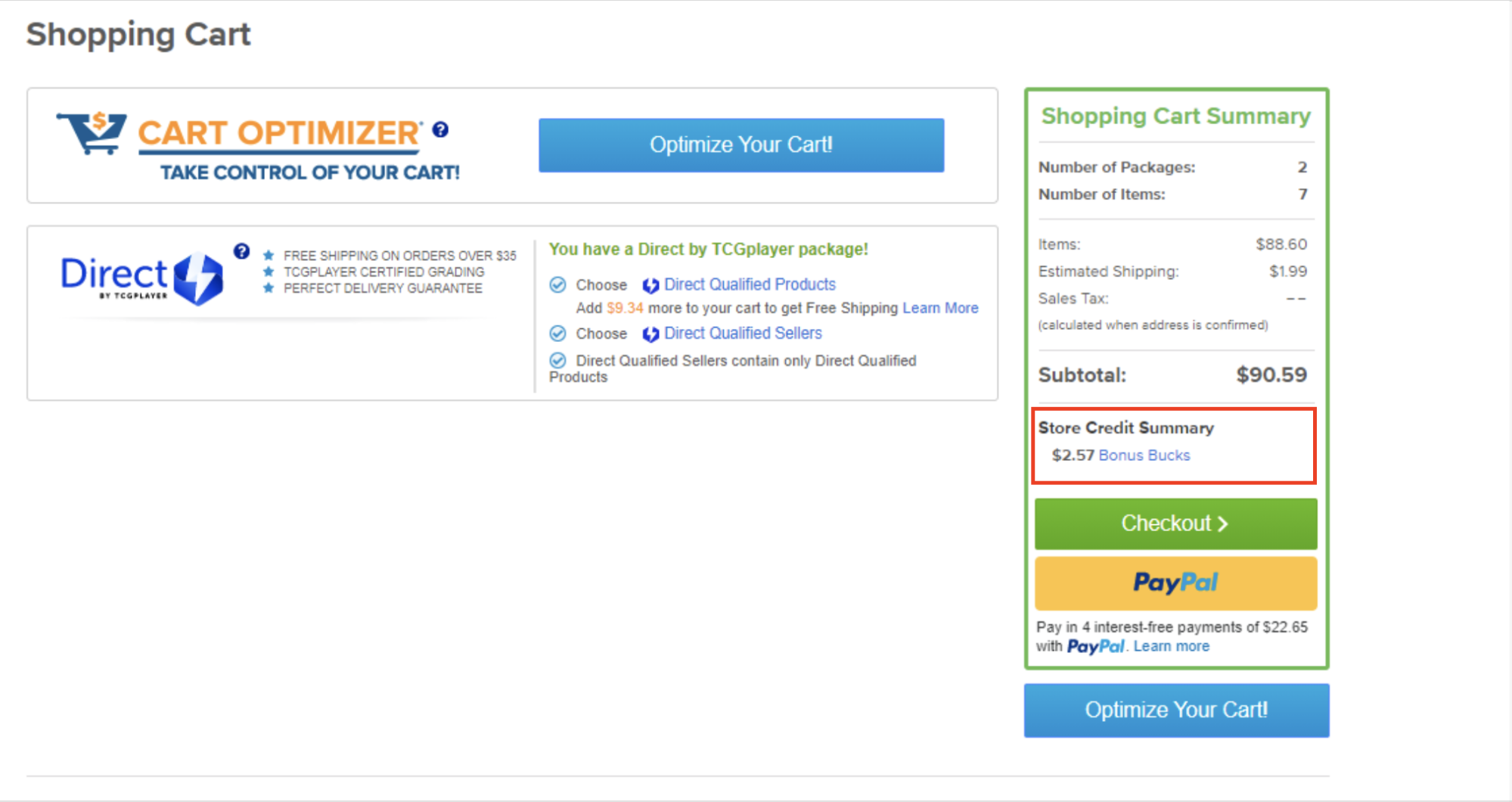Screenshot of an online shopping cart from a website for a company named "Direct," prominently featuring a blue and orange "Cart Optimizer" logo at the top. The text reads "Cart Optimizer: Take control of your cart." To the right, there's a large blue button with white text that says "Optimize Your Cart." Below this section, there's the Direct logo followed by text stating, "You have a Direct by TCGplayer package," with further details provided below.

In the right-hand column titled "Shopping Cart Summary," details are listed:
- Number of Packages: 2
- Number of Items: 7
- Items Total: $88.60
- Estimated Shipping: $1.99
- Sales Tax: $0.00
- Subtotal: $90.59

A red square highlights the "Store Credit Summary," specifying "$257 Bonus Bucks." Below this, there are buttons for "Checkout" and "PayPal" for completing the purchase.